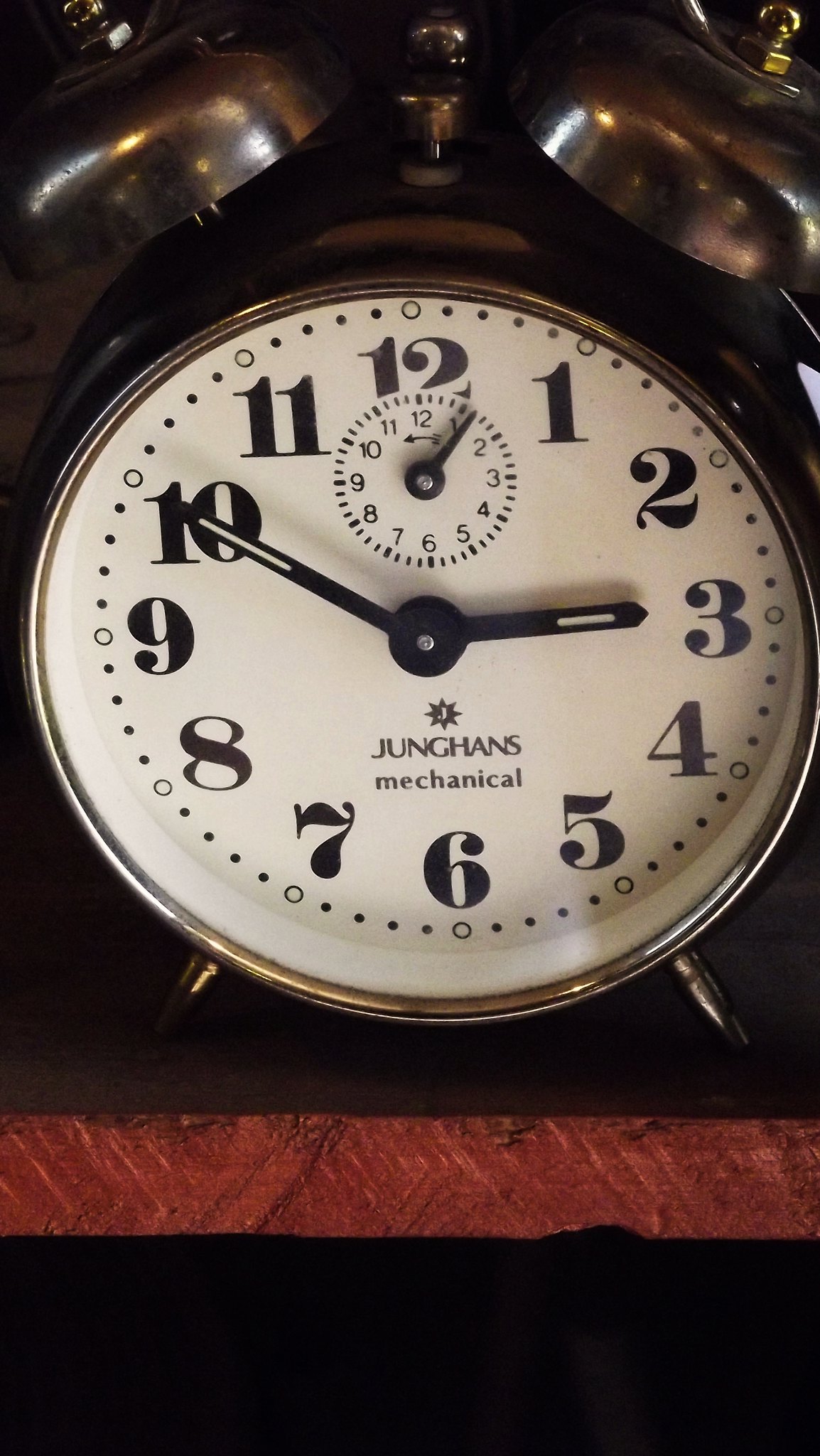The detailed color photograph showcases an old-style alarm clock resting on a wooden tabletop or shelf. The clock, approximately five inches in size, has a round body with a metallic black finish accented by a silver ring around its face. The white clock face features black numbers from 1 to 12, augmented by smaller black circles marking each minute. At ten minutes to three, the black hour hand points to the 3, while the longer minute hand is at the 10. Notably, the words "Junghans Mechanical" are inscribed beneath the hands. The clock's distinctive design includes two silver, disc-like bell ringers on top, resembling ears, and a smaller silver button in the middle. Additionally, it is supported by three angled rod-like legs that elevate it from the surface.